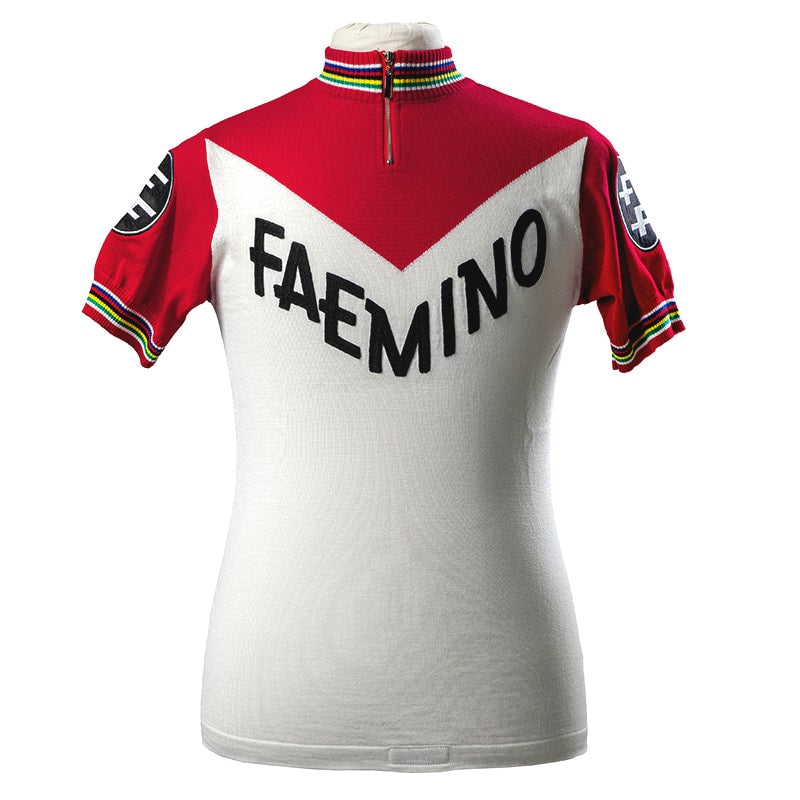The image depicts a vintage sports jersey displayed on a white fabric mannequin torso, with the neck clearly visible above the collar. The jersey is predominantly white on the lower portion, transitioning to red on the top section, reminiscent of a Marlboro packaging design with its distinctive V-shaped red point converging at the center of the chest. The collar features an encircling pattern of stripes in white, green, yellow, black, red, and blue, and it is equipped with a small, silver zipper with a black tab that is fully zipped up.

The jersey has short sleeves, with the sleeve ends similarly adorned with multicolored stripes. Notably, each sleeve bears a black circular patch, though the exact details within these patches are indiscernible. Across the chest, conforming to the V-shaped red design, are the bold, black letters spelling out "F-A-E-M-I-N-O." This well-fitted, form-hugging jersey merges a stark white lower half with a vivid, detailed upper segment, making it a striking visual piece on the mannequin.